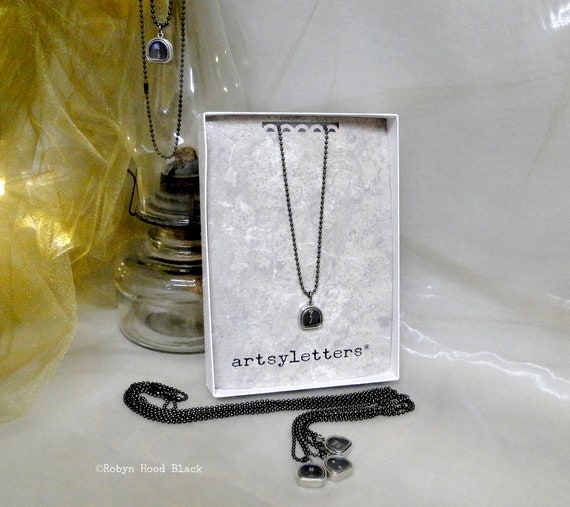The photograph features a detailed close-up of a jewelry display. Central to the image is a white box with a silver-gray interior, positioned upright to showcase a necklace inside. The necklace is made of small, millimeter-sized, steel-colored beads strung together forming a thin silver chain. It elegantly suspends a pendant with an almost oval shape, having a black center accented by a silver line through it. Below the pendant, inside the box, there's a small black text that reads "Artsy Letters," denoting the brand.

In front of the box, there are additional necklaces with similar thin chains and black pendants, arranged neatly on a white table with a marble-like surface. To the left, a slightly larger chain necklace is visible, mirroring the design but on a larger scale.

The background features a glass item, resembling an oil burner with a filament inside and a glass top and bottom, adding a decorative element to the scene. To the right of this, there is a piece of white sheeting, while on the left side, a see-through golden curtain is partially in view. Another necklace, larger and resembling the ones in the box, is draped near the top left corner, partially cut off by the frame. The overall setup is highlighted with a soft focus, emphasizing the jewelry's intricate details amidst its artistic environment.